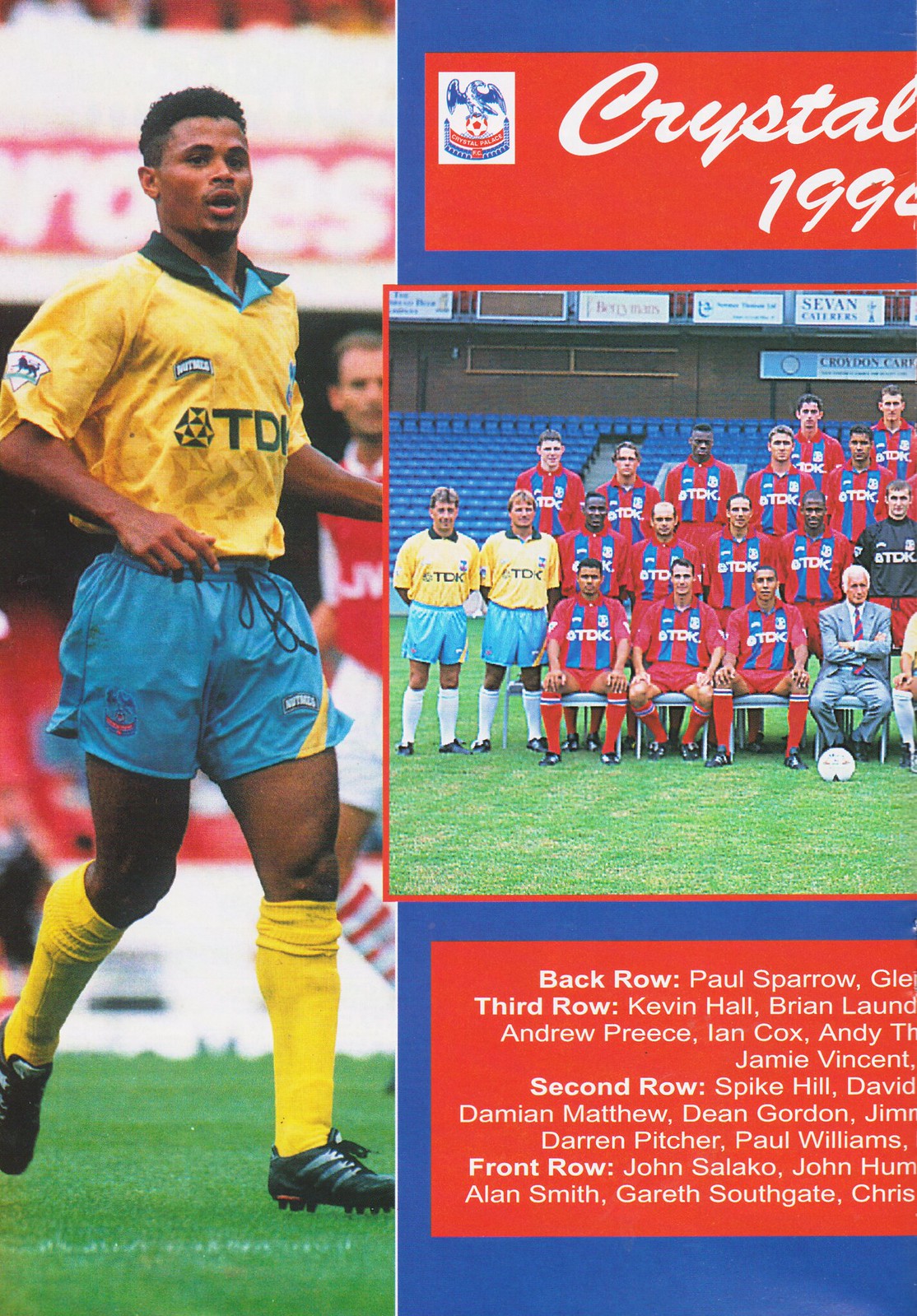This image is an advertisement or flyer for a soccer team. On the entire left side, there is a full-body shot of a black soccer player in mid-step run, with their mouth slightly open, on a green field. The player is wearing a yellow jersey with a tall folded-over blue collar, blue shorts with a yellow stripe on the left leg, yellow long socks, and black and gray soccer cleats. The yellow jersey features the letters "TDI" in green and some logos. To the right, there is a team portrait captioned "Bristol 1994" on a red background with white letters. The portrait shows multiple team members in red and blue jerseys; some are seated on chairs in the front while others are standing behind them, possibly on bleachers or chairs. At the very bottom, a red rectangle contains multiple lines of white font listing the players' names, including Paul Sparrow in the back row, Kevin Hall in the third row, Andrew Priest in the second row, and Spike Hill and Damian Matthew among others.